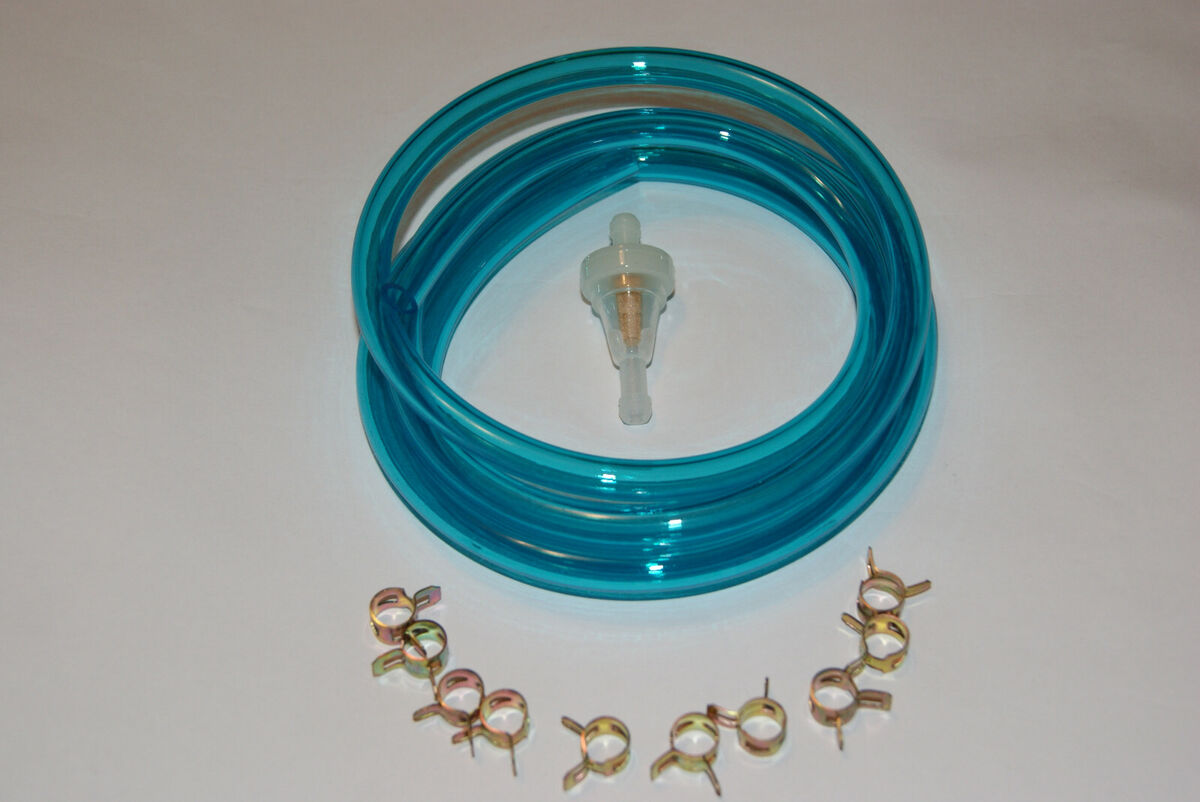In this horizontally rectangular photograph, there is a gray background featuring a prominent blue coiled pipe arranged in a circular manner. This light blue pipe, which appears to be transparent in some areas, is positioned centrally in the image. At the core of the coil is a semi-transparent white plastic nozzle, shaped somewhat like a top, with a small knob at the top and a larger end extending downward. This nozzle encloses a metallic, brownish-orange component that descends partway inside it and is intersected by a faint band.

Beneath the pipe on the gray surface are precisely 10 metallic clamps, primarily golden in color though a couple appear pinkish. These small clamps, each with two prongs, are scattered in a semi-circular pattern at the bottom of the image. The detailed arrangement includes the clamps oriented in various positions, with each prong pair situated close together. The overall scene is captured from an angle slightly above and to the side, adding depth to the composition.